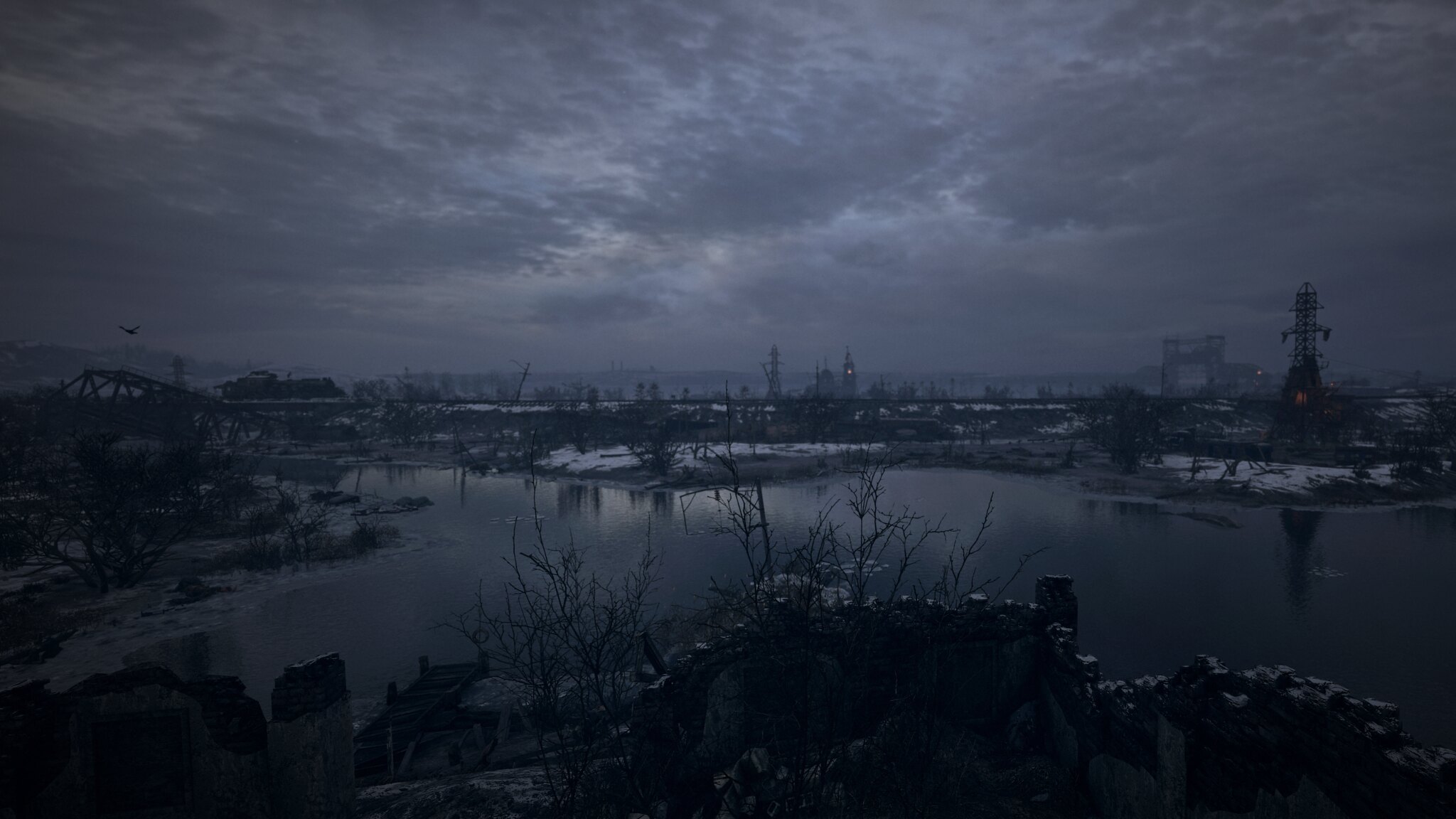This image, whether a highly detailed photograph or a screenshot from a video game, captures an industrial setting amid swampy or flooded terrain. The scene suggests a dilapidated area, possibly a town ravaged by time or conflict. Dominating the background is a tall metal tower—potentially a radio or construction tower—that rises impressively, reaching about 60% of the image's height. The color palette consists predominantly of dark blues and grays, enhancing the somber and abandoned atmosphere of the location. The clarity of the image highlights the intricate details of the waterlogged surroundings and the towering structure, evoking a sense of desolation and decay.